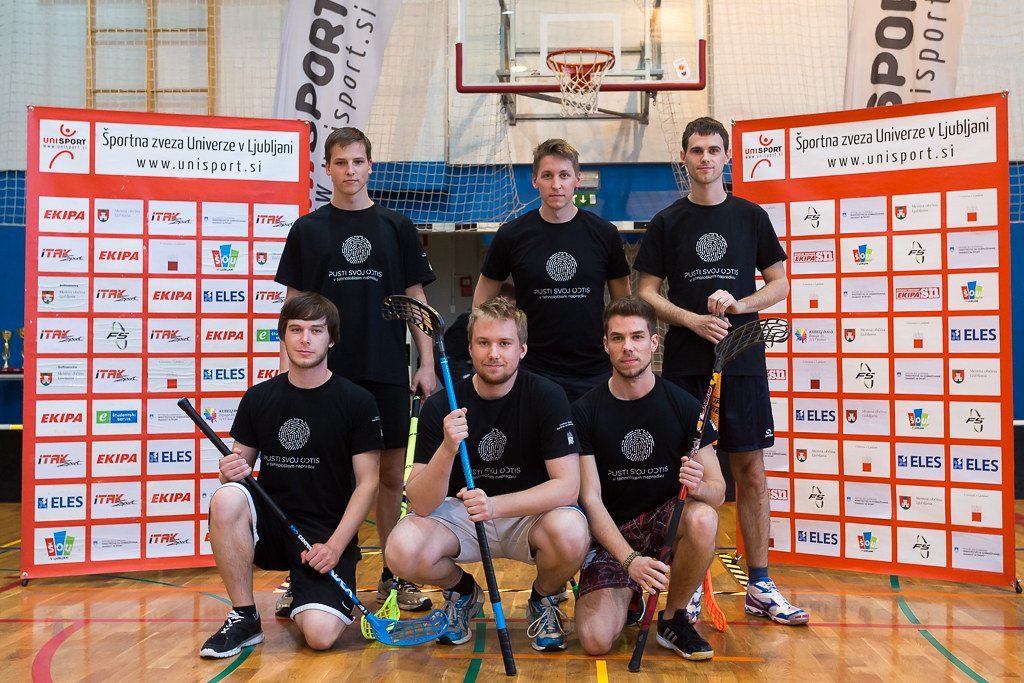The image features a team of six young men, likely a lacrosse team, posing for a photo inside a gymnasium. The players are arranged with three standing in the back and three squatting in the front, all holding their lacrosse sticks. The gym's background displays a basketball hoop and two large red sponsor boards filled with information and logos, predominantly in a language other than English, stating "Sportna Svesa Universi Ljubljani" and "www.unisports.si". The team members are uniformly dressed in black t-shirts adorned with a circular white logo and white fonts, paired with black shorts. Their sticks vary in color, including black and blue, orange, and red and black.